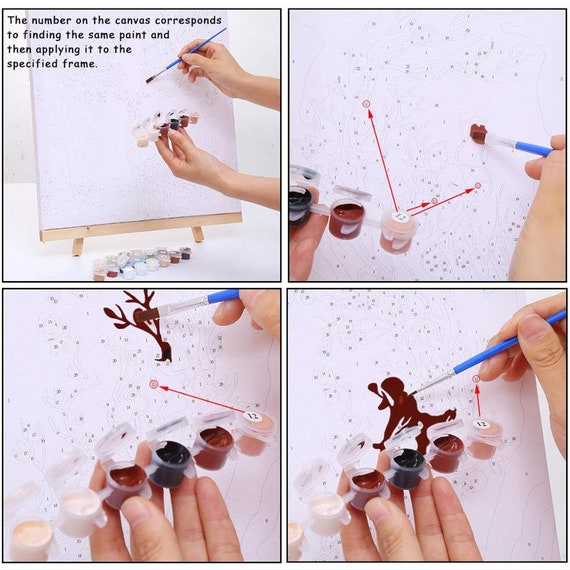The image is a panel comprising four distinct sections, each illustrating the step-by-step process of using a paint-by-numbers kit. In the top left, the first image shows two hands: the left one holding multiple small pots of paint and the right one holding a paintbrush. Displayed prominently on the blank canvas are faint, spattered dots, giving the impression of numbers that correspond to specific paint colors. The numbered guide informs that the number on the canvas matches a paint color to be applied to designated areas.

To the right, the second image zooms in on one such numbered area, specifically number 12, with a clear red circle highlighting this detail. Here, the artist has dipped the brush into the correctly labeled paint pot and has started to fill in the marked sections, making the relationship between the number on the canvas and the paint color evident.

The third section, located in the bottom left, continues this demonstration by showing more of the canvas being filled in, with number 12 paint now covering a larger area. The fourth and final image, in the bottom right, reveals a nearly completed section of the painting, emphasizing how the numbered guide leads to a cohesive and colorful artwork. The entire panel serves as a detailed and step-by-step visual guide on how to transform the initial grayscale spatter of dots and numbers into a vibrant and complete painting.